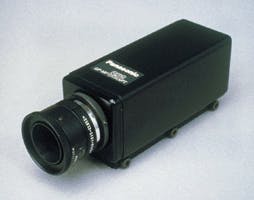This detailed photograph showcases a Panasonic charge-coupled device high-speed camera, shaped like a rectangular black box with a prominent round lens on the left side. The camera, which can capture images at high rates of either 30 or 60 frames per second, features a mix of black surfaces, white lettering for the label, and silver accents, especially around the lens which may serve as a zoom function. The device sits elevated on a small riser platform with three visible small black dots or screws at its base, set against a white background. The top bears the Panasonic logo, although it is somewhat difficult to discern. While neither buttons nor controls are visible in the presented angle, the overall design suggests it is from an older model, possibly from the late 70s to early 80s.